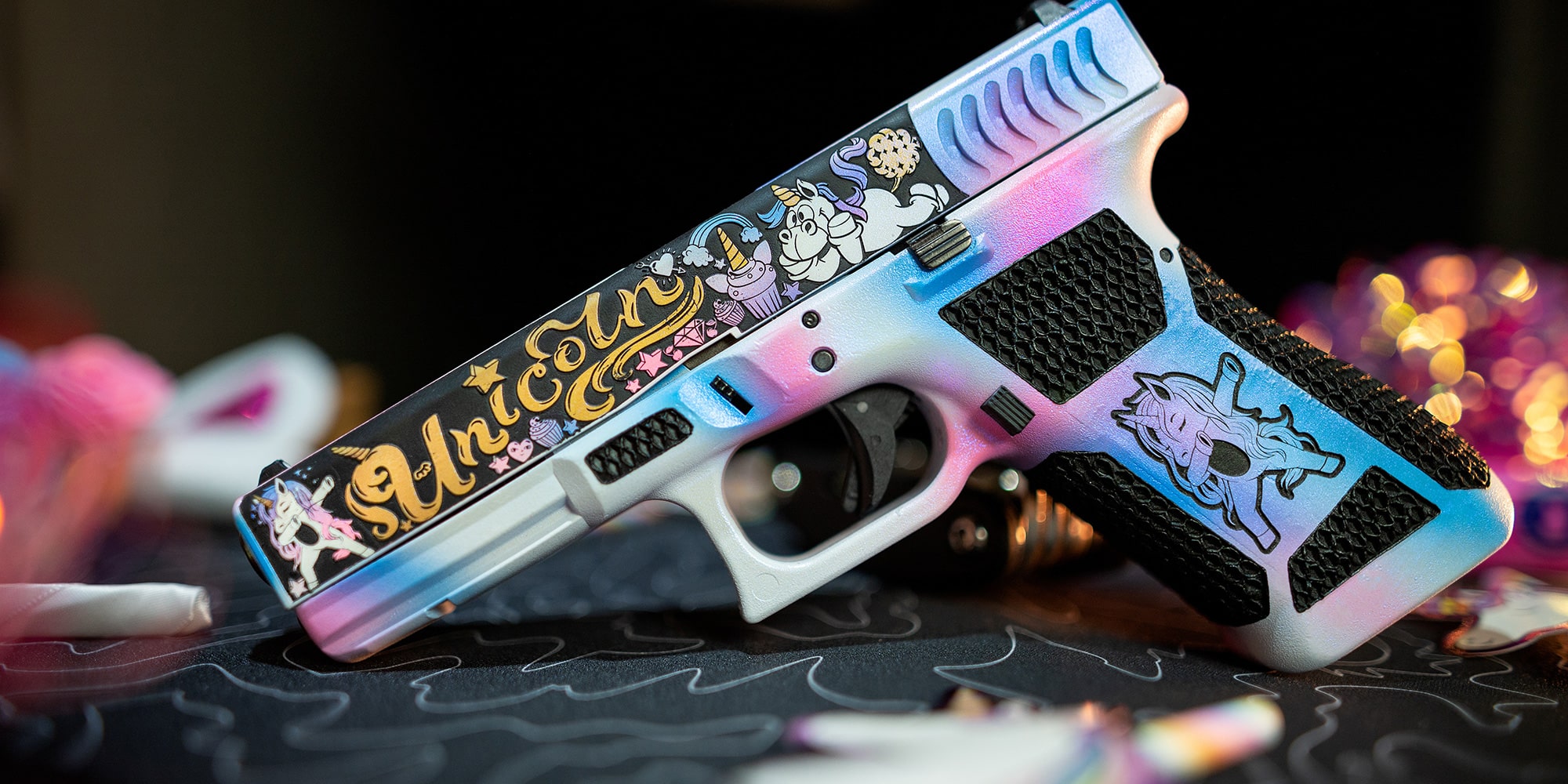This visually striking, artistically rendered photograph features a uniquely customized semi-automatic pistol. The gun is adorned with a variety of whimsical, unicorn-themed decorations. The color palette transitions through a prismatic gradient of pink, blue, and white. The barrel prominently displays the word "unicorn" in an ornate, cursive gold script, with a horn embellishing the 'U', a star dotting the 'I', and a swirl underlining the final letters. Various playful unicorn images embellish the piece, including a stylized unicorn standing or maybe dancing on the grip, a break-dancing unicorn, a cartoonish unicorn lying down with a flower, and another unicorn humorously depicted passing gas. The grip of the pistol is segmented into four parts of matte black rubber, contrasting with the pastel hues. The gun rests face down, barrel directed forward and to the left, the butt to the right, on a black fabric background featuring white squiggles which provide a stark contrast that accentuates the bright, colorful design of the pistol. The overall scene is washed in a mix of bright colors with a prominently black, contrasty area that brings attention to the gun's vivid and imaginative decorations.